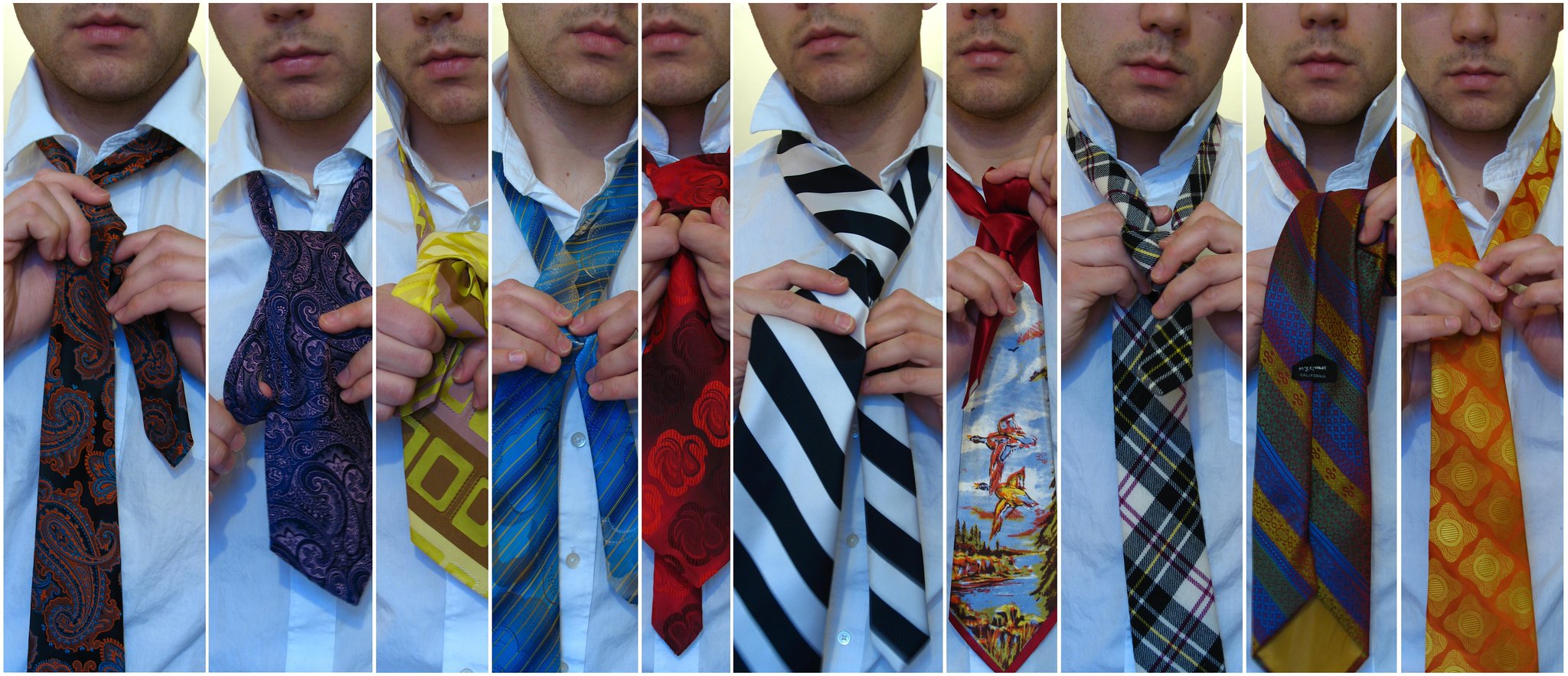This photograph showcases a series of 10 close-up images of a young man, depicted from his nose to his waist, all aligned side-by-side. He is wearing a white collared shirt, which remains unbuttoned at the top, revealing a glimpse of his facial hair with a slight shadow on his chin. Each panel captures him at various stages of tying different ties, creating a collage effect. The ties, each distinct in design and color, include:

1. A dark red and green paisley tie.
2. A blue paisley tie.
3. A yellow and brown bandana-like tie.
4. A blue striped tie with light and dark blue tones.
5. A red tie adorned with roses.
6. A black and white striped tie.
7. A tie featuring birds, mountains, and water.
8. A black, white, and red plaid tie.
9. A yellow and navy blue striped tie.
10. An orange and gold checkered tie with small diamond patterns.

The expressions on his face vary slightly across the images, and the ties are at different stages of being tied, highlighting the meticulous process of achieving the perfect knot.